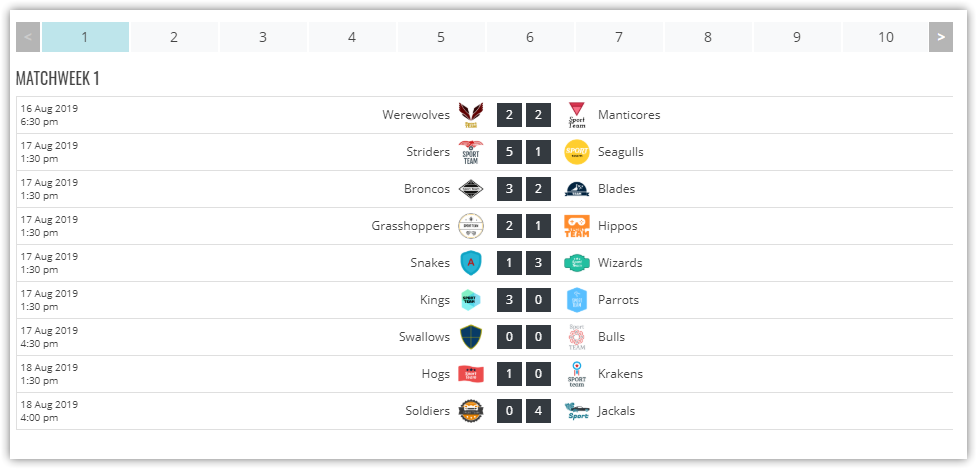The image showcases a detailed schedule of sports scores, organized by match week and date. At the top left, the title "Match Week 1" is prominently displayed, with the current week highlighted in blue, while the subsequent weeks (2 through 10) are listed to the right and shaded in gray. Below, there is a chronological list of match times and dates. The first match is scheduled for August 16, 2019, followed by six matches on August 17, and concluding with two matches on August 18. Each game is listed with the competing teams on the left and right, respectively, with the scores displayed in black squares centrally aligned between the team names. The entire schedule includes nine total games, arranged in a vertical column with thin horizontal lines separating each matchup. The background of the image is white, framed by a gray border.